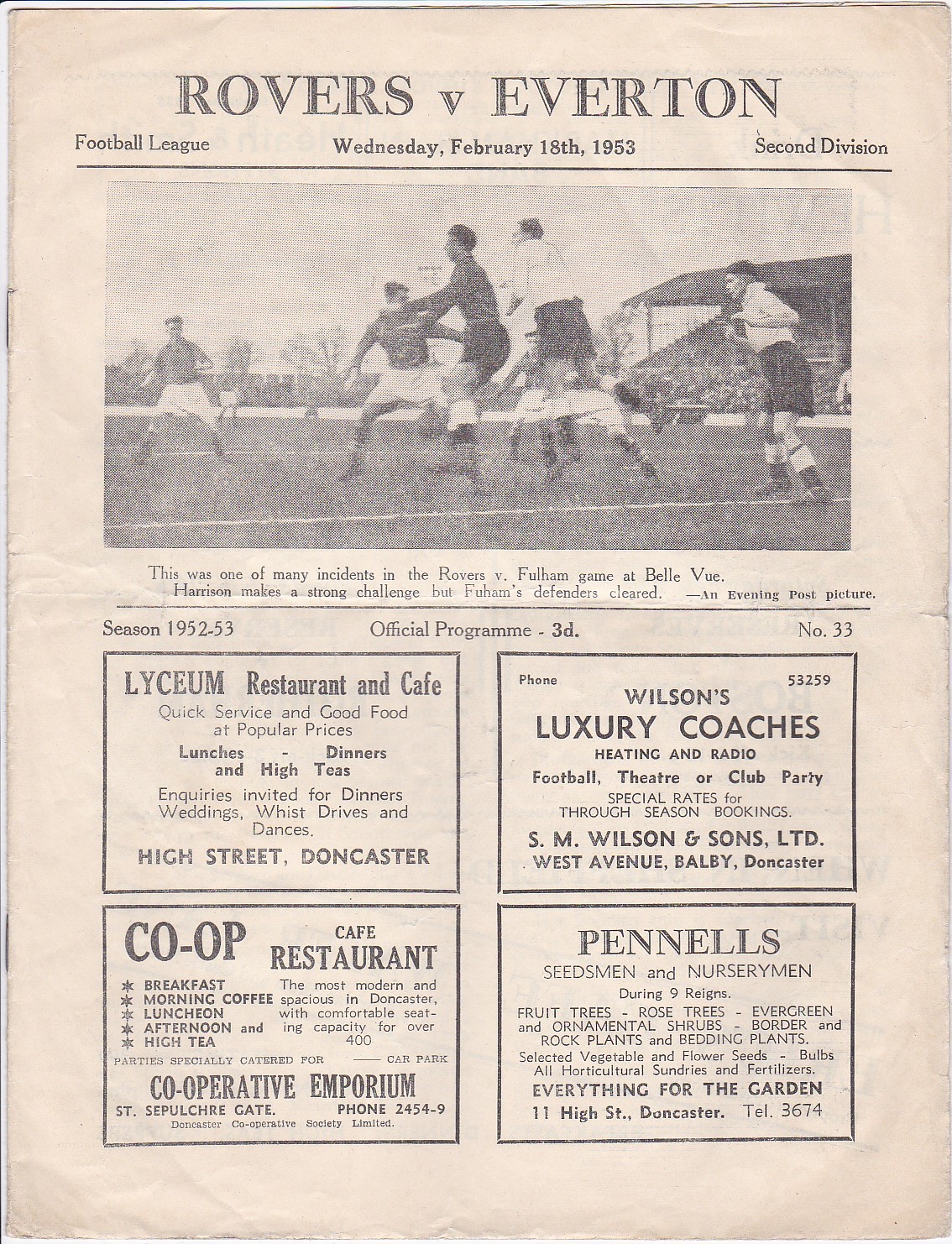This image captures an old, weathered scan of a sports article or publication, likely an official program for a football (soccer) match. The cover, now more brown than white with age, reads "Rovers vs. Everton Football League, Wednesday, February 18th, 1953, 2nd Division". Dominating the middle is a black and white photograph of players engaged in the game, though the low quality and age make it hard to discern details. Below the picture, a caption states, "This was one of many incidents in the Rovers vs. Fulham game at Bellevue. Harrison makes a strong challenge, but Fulham's defenders cleared. An evening post picture." The program, labeled "Season 1952-53, Official Program 3D, Number 33," features four advertisements on the lower half. These include: Lyceum Restaurant and Cafe offering quick service and good food at popular prices, Wilson's Luxury Coaches with heating and radio for football, theater, or club parties, Co-op Cafe Restaurant, and Pinnell's Seedsmen and Nurserymen.